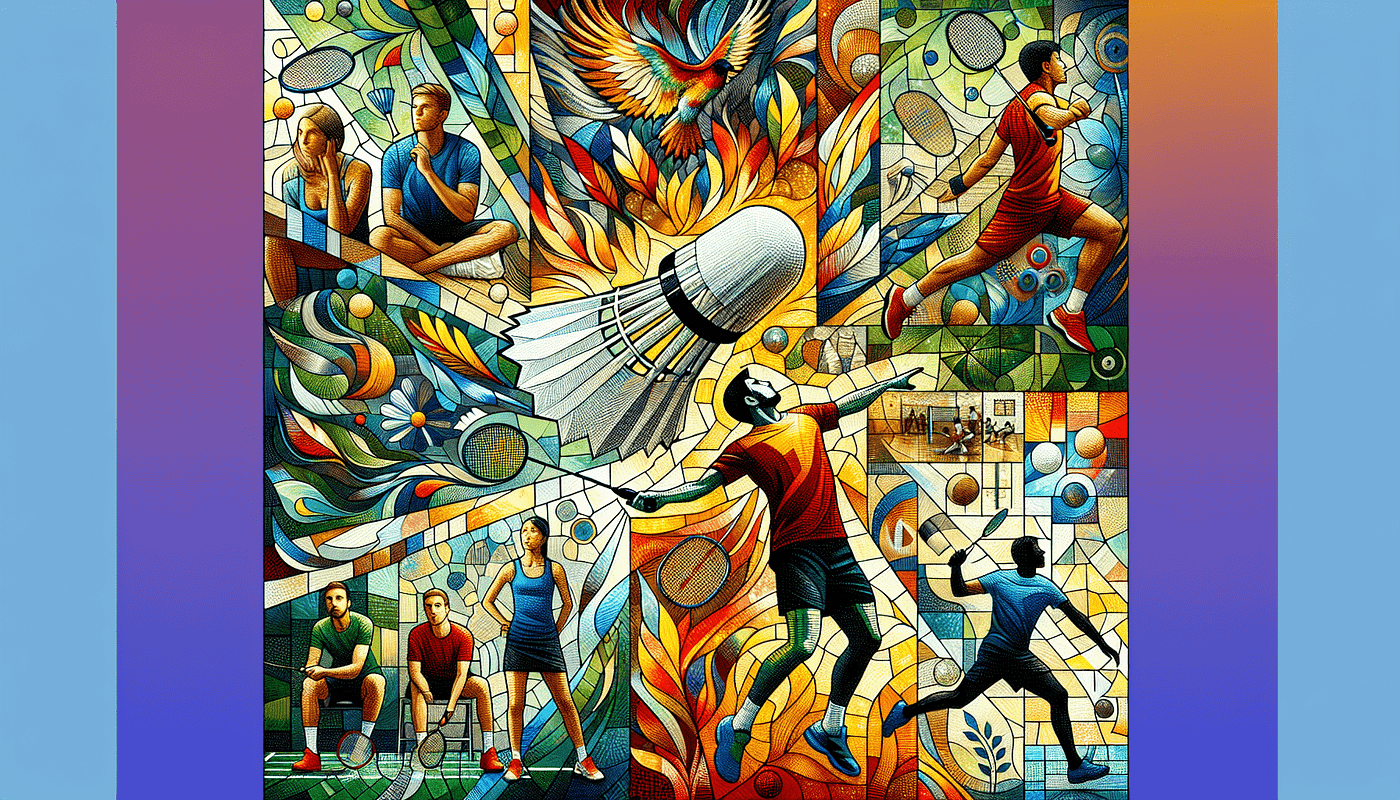This vibrant and intricate image is a stained glass montage themed around badminton, boasting a rich array of colors including reds, blues, greens, and yellows. The artwork is divided into several panels, each brimming with detailed scenes and vivid hues, creating a mosaic-like effect reminiscent of church windows.

Starting from the top left, there is a depiction of a man and a woman seated in a thoughtful pose, seemingly contemplating a badminton match. Adjacent to this scene, a vibrant bird soars above a shuttlecock, adding a dynamic element to the tableau. Next, a figure is shown running amidst a backdrop of badminton rackets, conveying a sense of motion and activity.

Below these panels, there is a smaller depiction of individuals actively engaged in a game of badminton. To the right of this, a silhouette of a player mid-action captures the sport’s energetic spirit. Continuing clockwise, a person wearing an orange shirt is vividly portrayed in the midst of playing badminton.

The overall composition includes seven to nine panels, each meticulously crafted to illustrate various aspects of the sport. Central to the artwork is an ornate depiction of a shuttlecock, surrounded by players in various stances associated with the game. In the bottom left, men holding rackets are seated, perhaps preparing for a match. The entire scene is accentuated with yellow and red leaves under the colorful bird, which adds a thematic continuity and balance to the piece.